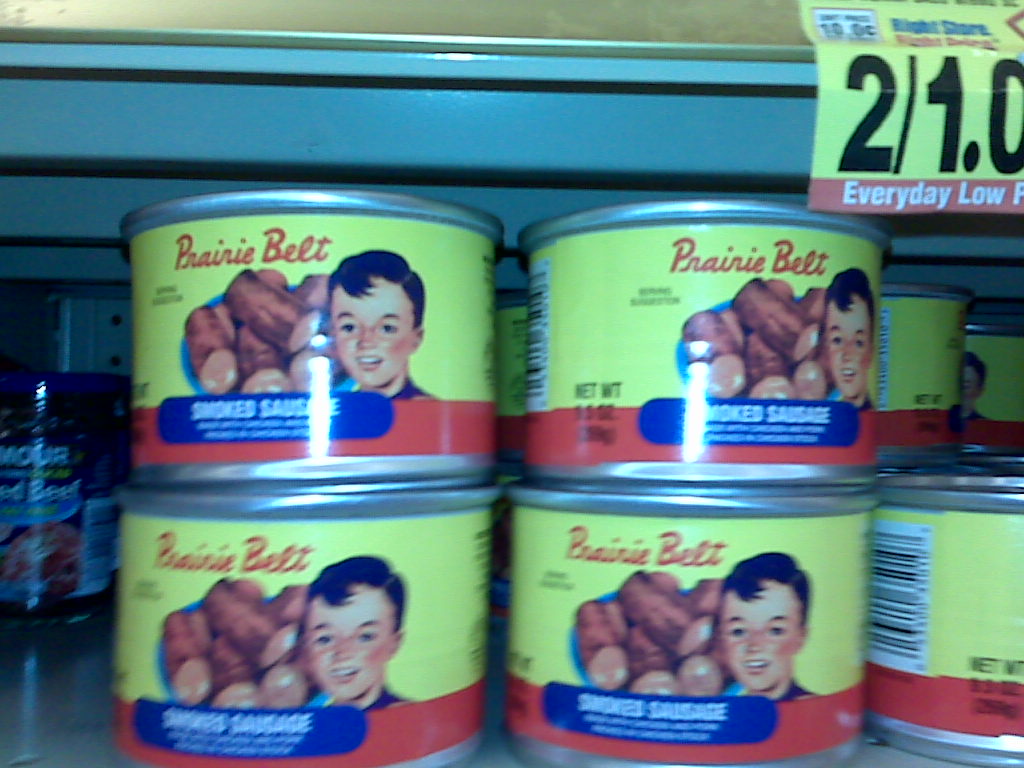This color photograph, taken inside a grocery store, presents a detailed view of an aisle shelf displaying small cans of Prairie Belt smoked sausages. Each can is vibrantly designed with a yellow and red label accented with blue and measures approximately 3.3 ounces. Dominating the label is an illustration of a young boy, around five or six years old, with short dark hair, freckles, and brown eyes, shown with his mouth open. Next to him is a blue plate or bowl filled with about five or six smoked sausages, emphasizing the product inside. A sign above the cans advertises an everyday low price of two for a dollar. The shelf is stacked with many cans, arranged at least two high. To the left of the Prairie Belt cans, there is a glass jar of Armour Brand corned beef, adding context to the grocery store setting. Despite some blur in the photograph, the primary details of the boy, the sausages, and the brand name "Prairie Belt" are clear and striking.